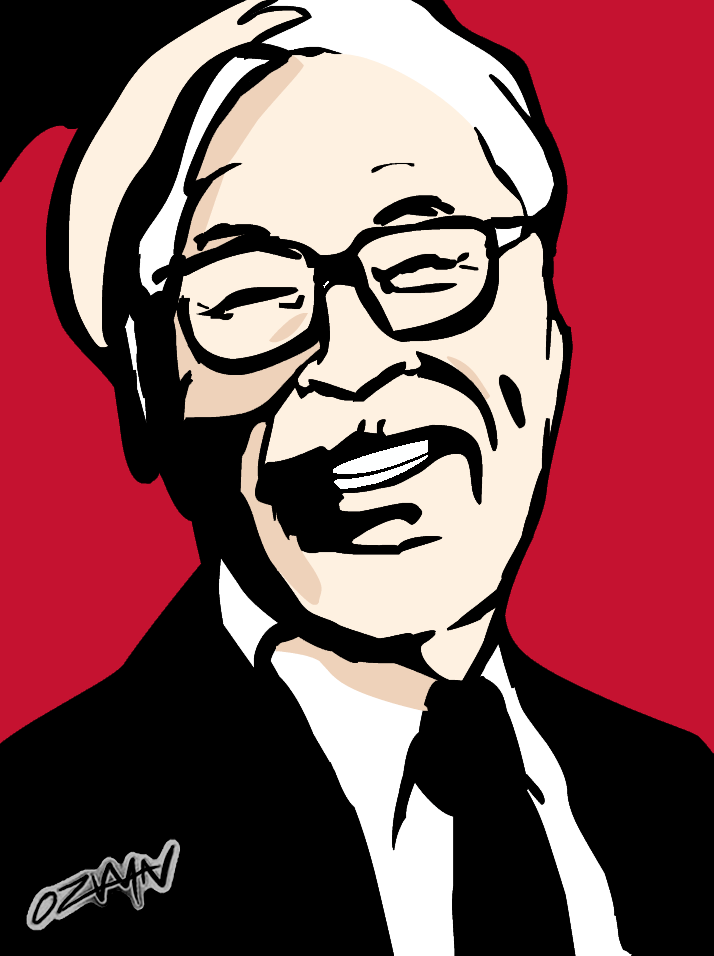This color graphic artwork features an Asian man smiling warmly, depicted from the head and shoulders. Employing a palette of red, white, black, and pale beige pink tones, the artist presents the figure in a style that leans towards abstract. The man is turned slightly to the left, gazing directly at the viewer through black-framed glasses that sit above his crinkled eyes, emphasizing his genuine smile. His white hair contrasts distinctly against the vibrant red background. He is dressed sharply in a white dress shirt, black tie, and black jacket. Deep, expressive lines trace from his nose to his mouth, highlighting the joy in his expression. The heavy lines and color choices give the piece a resemblance to an Andy Warhol composition, with some viewers noting an initial impression akin to the Kentucky Fried Chicken Colonel Sanders mascot. The bottom left corner of the piece is signed with "OZ" and what appears to be "MN." The overall aesthetic, with its bold, simple colors and thick lines, imparts a strong visual impact.